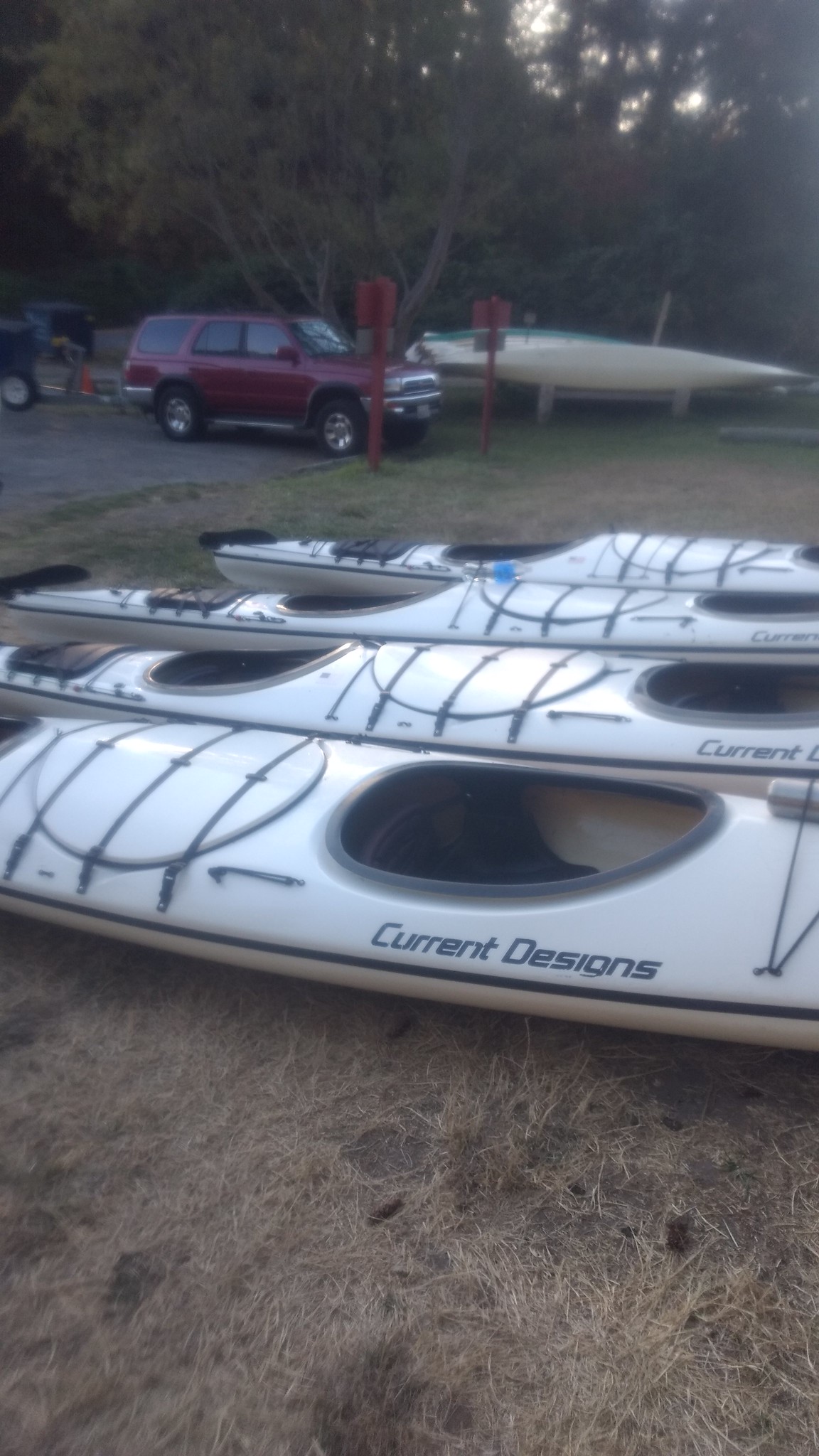The outdoor daytime photograph, taken under hazy or low light conditions and slightly out of focus, prominently features three two-person white kayaks arranged mostly horizontally, with only their central sections fully visible. The kayaks, marked with "Current Designs" in blue lettering, have oval openings and some dried grass scattered over them, resting on a dirt foreground. To the right, a maroon or purple Bronco with a boat trailer behind it is captured in a three-quarter view, and nearby, a yellow and green boat is visible. The background showcases trees with varying shades of green leaves, and sunlight peeks through them. There are also two indistinct signs and potentially another vehicle or object partially seen in the distance.